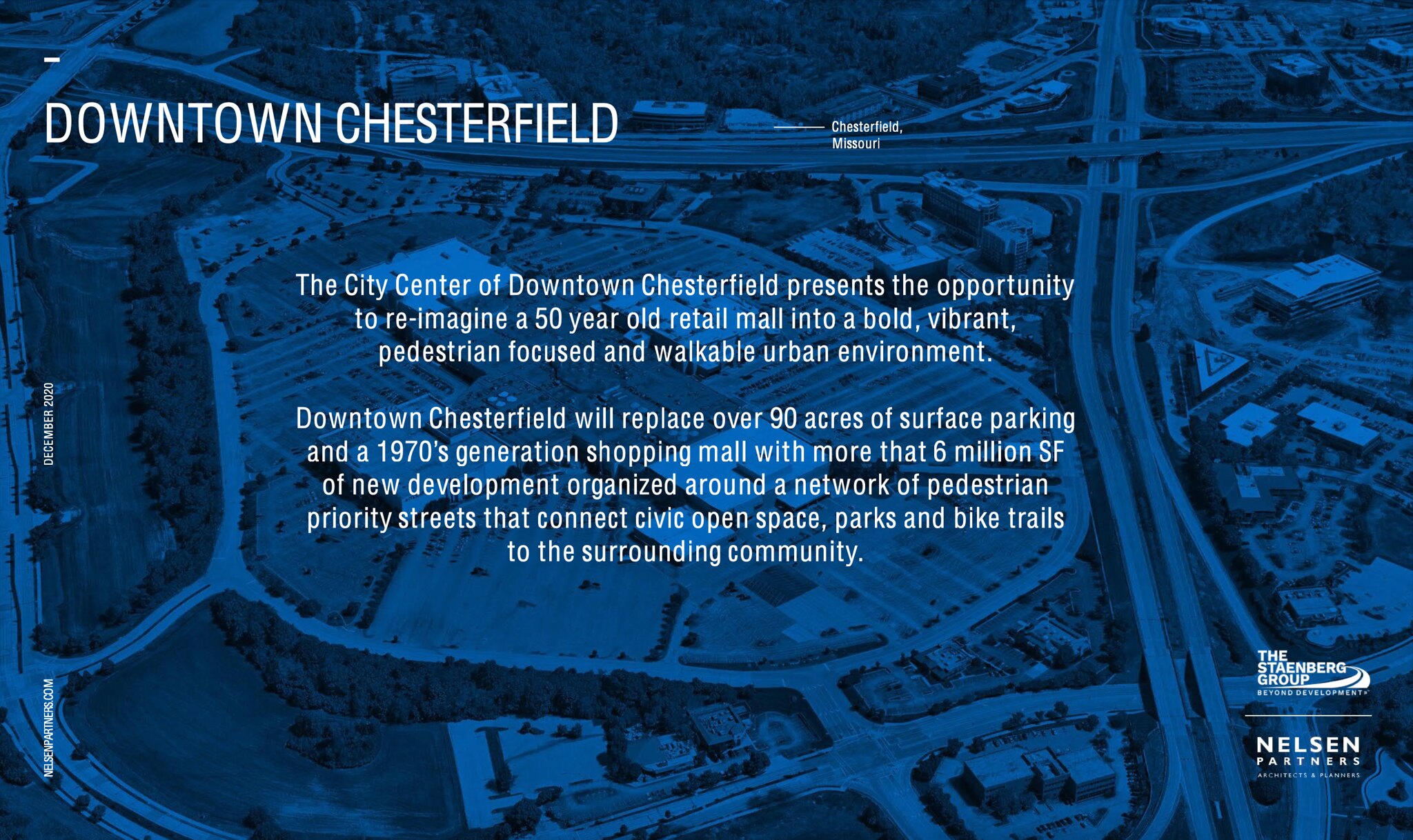The image is an aerial view, tinted in shades of deep blue, depicting a cityscape with a network of buildings and roadways crisscrossing through the area. Central to the image is a large circular zone that serves as a focal point, with roads leading into it. Overlaying the image is white text, prominently positioned in the upper left-hand corner, which reads, "Downtown Chesterfield." Further centered text elaborates, "The City Center of Downtown Chesterfield presents the opportunity to reimagine a 50-year-old retail mall into a bold, vibrant, pedestrian-focused, and walkable urban environment. Downtown Chesterfield will replace over 90 acres of surface parking and a 1970s-generation shopping mall with more than 6 million square feet of new development. This development is organized around a network of pedestrian-priority streets connecting civic open spaces, parks, and bike trails to the surrounding communities." In the lower right-hand corner, two logos are visible, representing the Steinberg Group and Nelson Partners. The overall composition suggests plans for a significant urban redevelopment project aimed at transforming the outdated mall into a vibrant, community-centered environment.